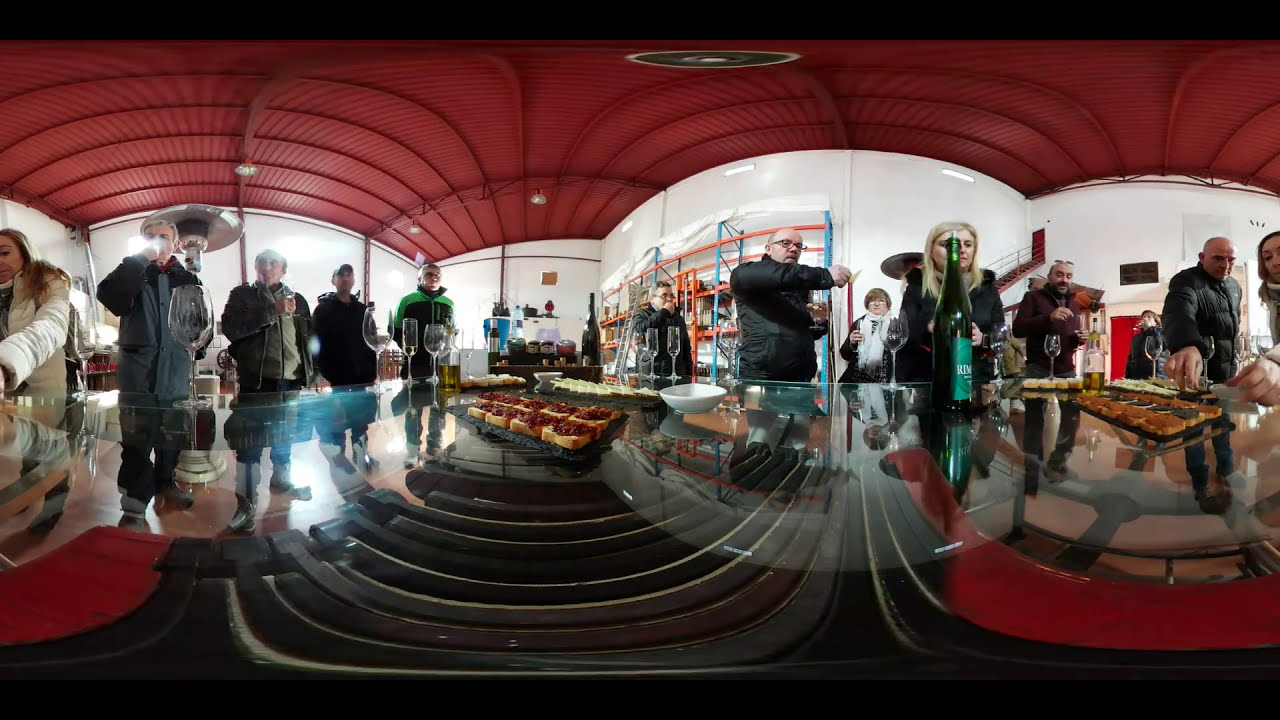In this vibrant color photograph taken from a countertop, a bustling food station is the focal point. The countertop is laden with several trays of food items, including an assortment of pastries and toast topped with various spreads. Several empty glasses and a bottle of champagne with a cork in it sit among the trays. To the left, several people, clad in jackets suggesting a chilly environment, are reaching for the food, while others are either drinking from or holding wine glasses. In total, around thirteen people are seen mingling, with some savoring the pastries and others holding food. The room features a striking contrast with a bright red ceiling adorned with slats of wood and a stark white wall behind the countertop. Adding a splash of industrial aesthetic, there is orange and blue scaffolding in the background. A red door to the right completes the vivid scene. Reflections of the red ceiling can be noticed on reflective surfaces in the lower third of the photo, hinting at a possible red carpet or tiled floor.